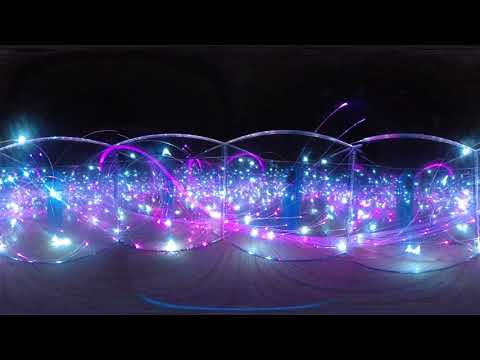This image depicts a visually striking array of tiny lights, resembling a specialty Christmas display, against a consistent black background. The photograph is framed vertically with a black stripe on the top and bottom, accentuating its rectangular shape. The lights, intricately bunched together, are woven into a dark or possibly light gray cloth that shows discernible ridge lines. These lights exhibit a soft, enchanting glow in shades of purple, blue, white, and some dark blue, creating an almost swirling pattern, and are structured in four distinct sections separated by vertical wires. Each section has a central blue light surrounded by more subtle purple hues, giving the entire display a luminous and organized appearance. Specks of white, likely bulbs, interspersed with purple and white lines, further enhance the mesmerizing effect. The overhead presence of four white arches adds a touch of elegance, merging to form an intricate pattern against the dark background.